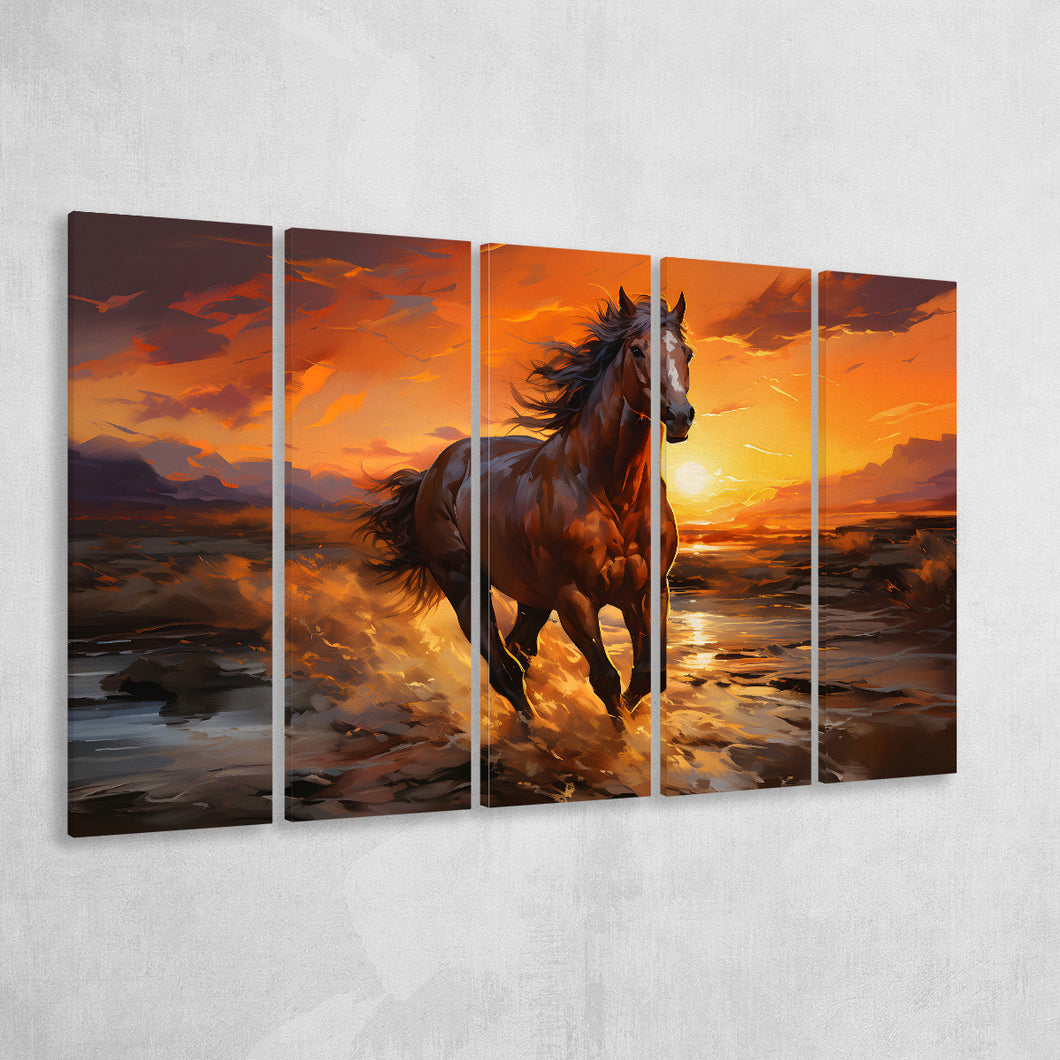The image displays a segmented painting on an off-white wall, divided into five long vertical frames that collectively form a single unified scene. The artwork depicts a powerful, brown horse with a white streak down the middle of its face, galloping towards the viewer through a shallow body of water. As the horse rushes forward, its strong muscles and beautiful mane are prominently visible. The background transitions from a vibrant yellow sunset to a deeper, orange-hued sky, with clouds scattered overhead. The sun, low on the horizon, casts a warm glow that reflects on the water around the horse, enhancing the dynamic and vivid atmosphere of the scene.